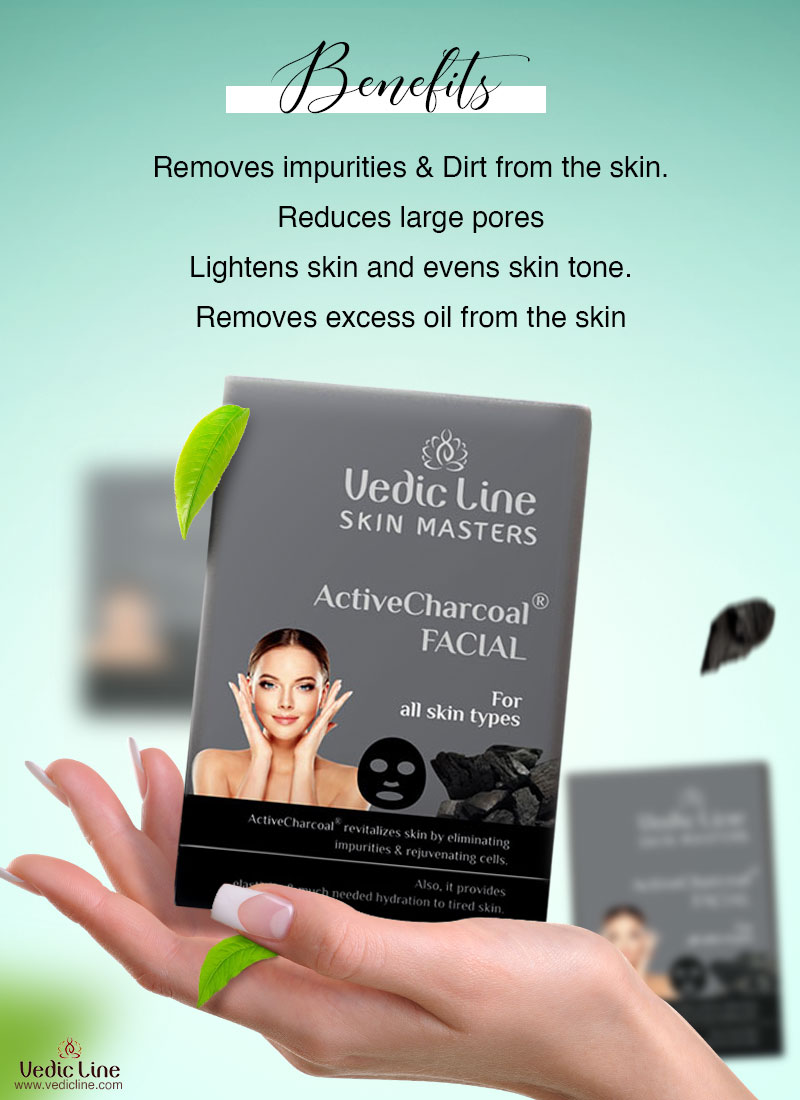This vertical rectangular advertisement showcases the Vedic Line Skin Masters Active Charcoal Facial prominently at its center. Set against an aqua-colored background, the product—a gray box with black lettering—features a small picture of a woman with her hair pulled back, her hands near her face. Above the product, a white triangle sits with the word "Benefits" inscribed through it in black print, detailing the product's capabilities: removes impurities and dirt from the skin, reduces large pores, lightens the skin and evens skin tone, and removes excess oil from the skin. The box, also showing the text "for all skin types," rests delicately in a woman's hand, adorned with long, polished fingernails. A green leaf hangs off the box, with another leaf on one of her fingers. The bottom left corner of the image features the text Vedic Line and the website www.vedicline.com. Behind the main product, subtle, blurred images of the product add depth to the composition.